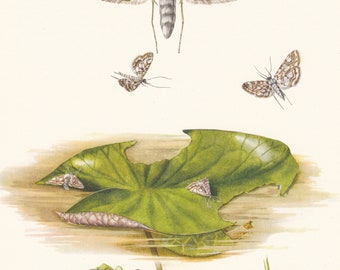The image is a detailed drawing or painting with a square shape and a beige background. Dominating the lower two-thirds of the composition is a large green leaf, possibly a lily pad, that lies flat on a surface resembling a wooden floor with brown streaks. The leaf exhibits intricate vein details and has browned, curling edges with three large, bite-like holes. Surrounding the leaf, various insects, including moths and butterflies, are depicted. Some insects are perched on the leaf, appearing to feed on it, while others hover above. Notably, two moths with brown speckled wings are flying slightly above the leaf, creating a dynamic scene. Towards the top of the image, part of a larger insect is visible—a portion of its body, gray and white striped tail, and legs can be seen hanging down, suggesting it is partially cut off by the frame’s edge. The overall scene is teeming with life and intricacy, capturing a moment in nature with remarkable detail.